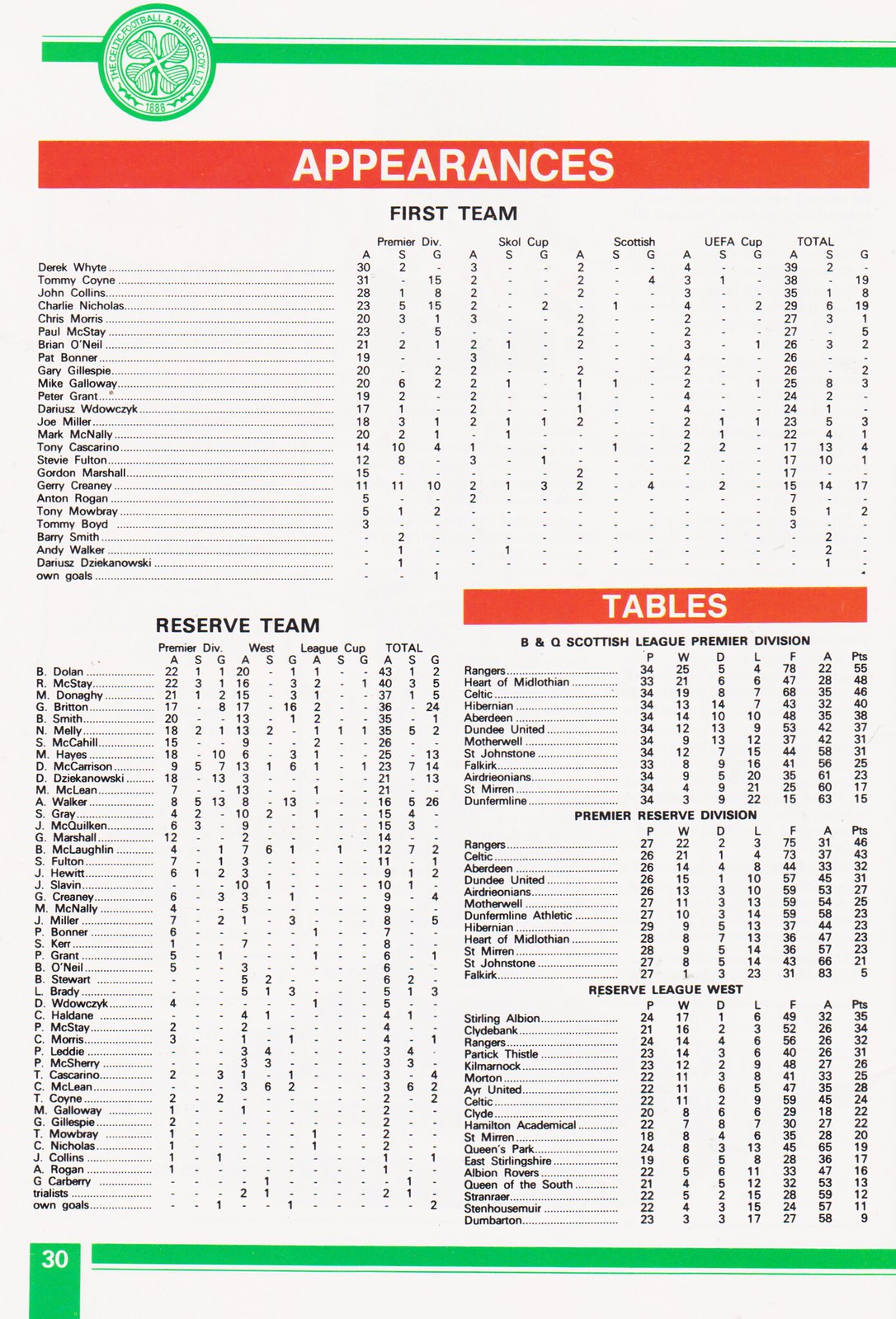The image is a detailed page from a magazine, designated as page 30, concerning British football statistics. The page is primarily white with a distinct green line at the top and a logo with a shamrock on the left side. Beneath the logo, there's a red rectangle labeled "Appearances" in white text. This section is divided into two parts: "First Team," which lists player names and their statistics across various competitions, including Premier Division, Skol Cup, Scottish Cup, UEF Cup, and total appearances; and "Reserve Team," which similarly catalogues player names and their corresponding statistics. On the right side, another red rectangle labeled "Tables" in white text presents standings for different divisions, namely the Scottish League Premier Division, the Premier Reserve Division, and the Reserve League West. The font throughout is noted to be very small, contributing to the densely packed information on the page.